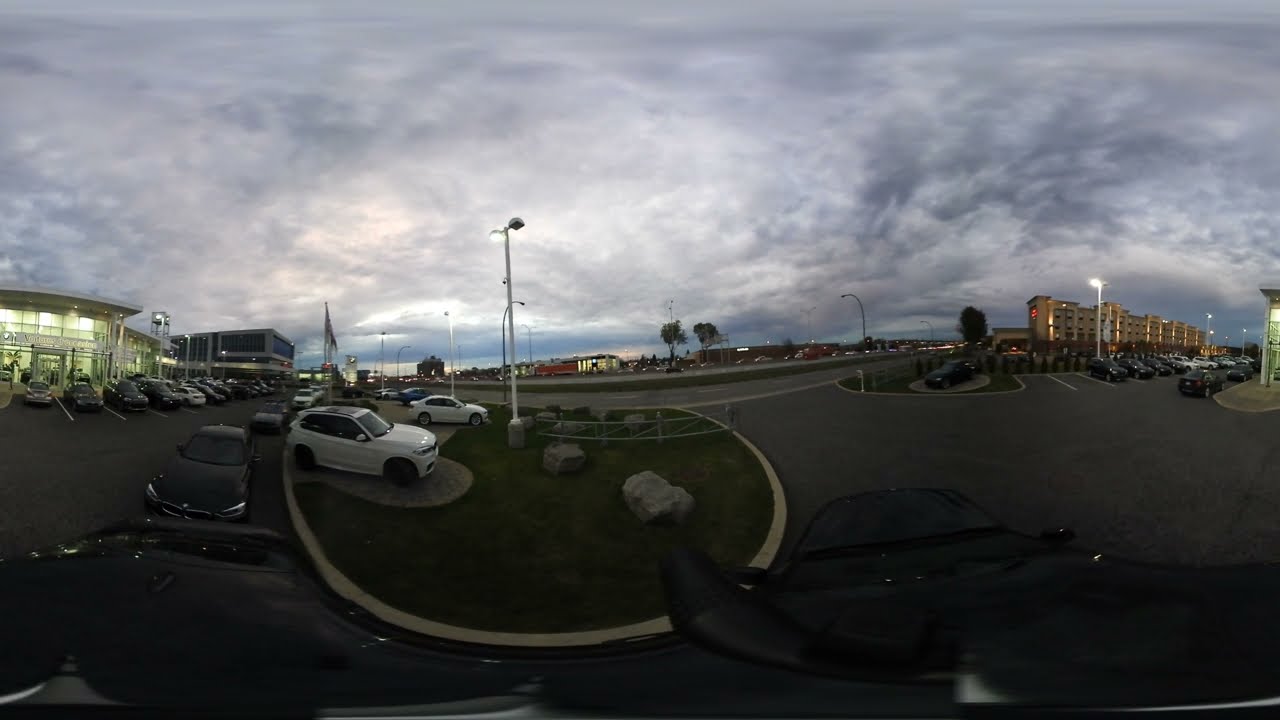This photograph captures an outdoor scene in a parking lot on a stormy day, likely taken from inside a car as evidenced by the presence of a vehicle's interior at the bottom of the image. The image is characterized by the distinctive distortion of a fisheye lens effect, which bends and stretches the scene into a broad, encompassing view. 

To the right, there is a large building, possibly a hotel, with numerous cars parked in front. The left side of the image features a couple of buildings, with one brightly illuminated and another in darkness, suggesting it might be a shopping center. Central to the parking lot is a rounded grassy area, landscaped with large rocks, streetlights, fencing, and several parked cars, including two prominent white subcompact cars on the left. 

The sky overhead is filled with dark, stormy clouds, though a patch of lighter sky and hints of blue are visible towards the center. The lamps are on, indicating either late evening or early morning, as the sun is low. Surrounding the parking lot, there are streets leading off to the left and right, flanked by more buildings in the background and a few trees scattered throughout. The image’s fisheye effect gives it a slightly surreal and all-encompassing feel.